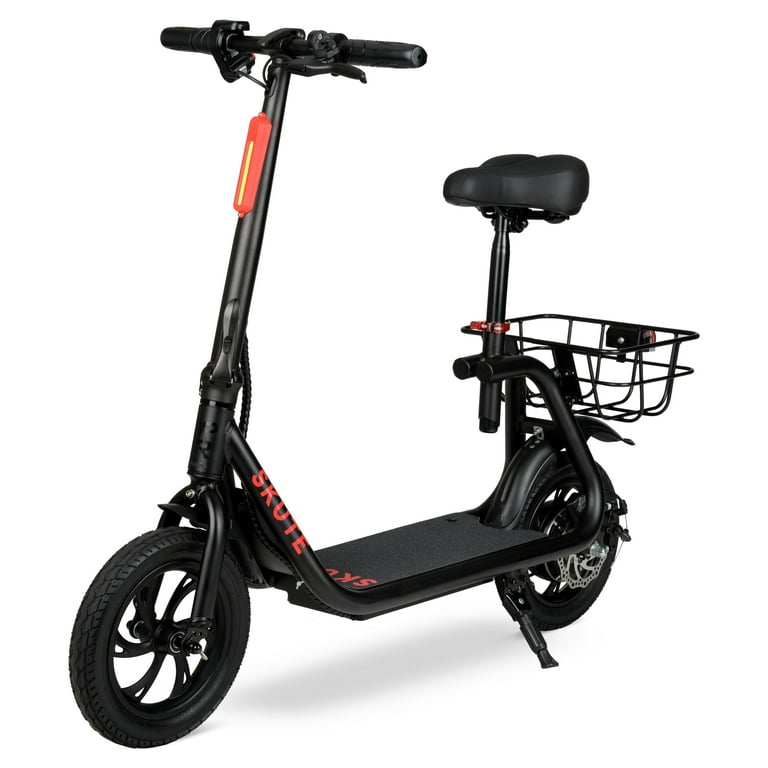This image is a detailed photograph of a black electric scooter set against a blank white background, likely outdoors. The scooter features a typical bike-style seat, supported by a rod, with a basket positioned on its back end. It has two wheels and includes standard elements such as a fender on the back and a kickstand to prop it up. The handlebar is equipped with a brake mechanism and has distinctive red accents, including a red cylinder atop the stem. The tube connecting the stand to the handlebar features the letters "S-K-O" and partially readable "T-E" in red, suggesting the brand name "SKUTE."

Additionally, there's a red trim along the footrest area, and a red light or reflector mounted on the front of the scooter. This sit-down scooter has a throttle on the left handlebar and a mounting bracket on the right. The light source is directly overhead, providing a clear, unfiltered view of the scooter's predominantly black frame, with the red highlights standing out prominently.